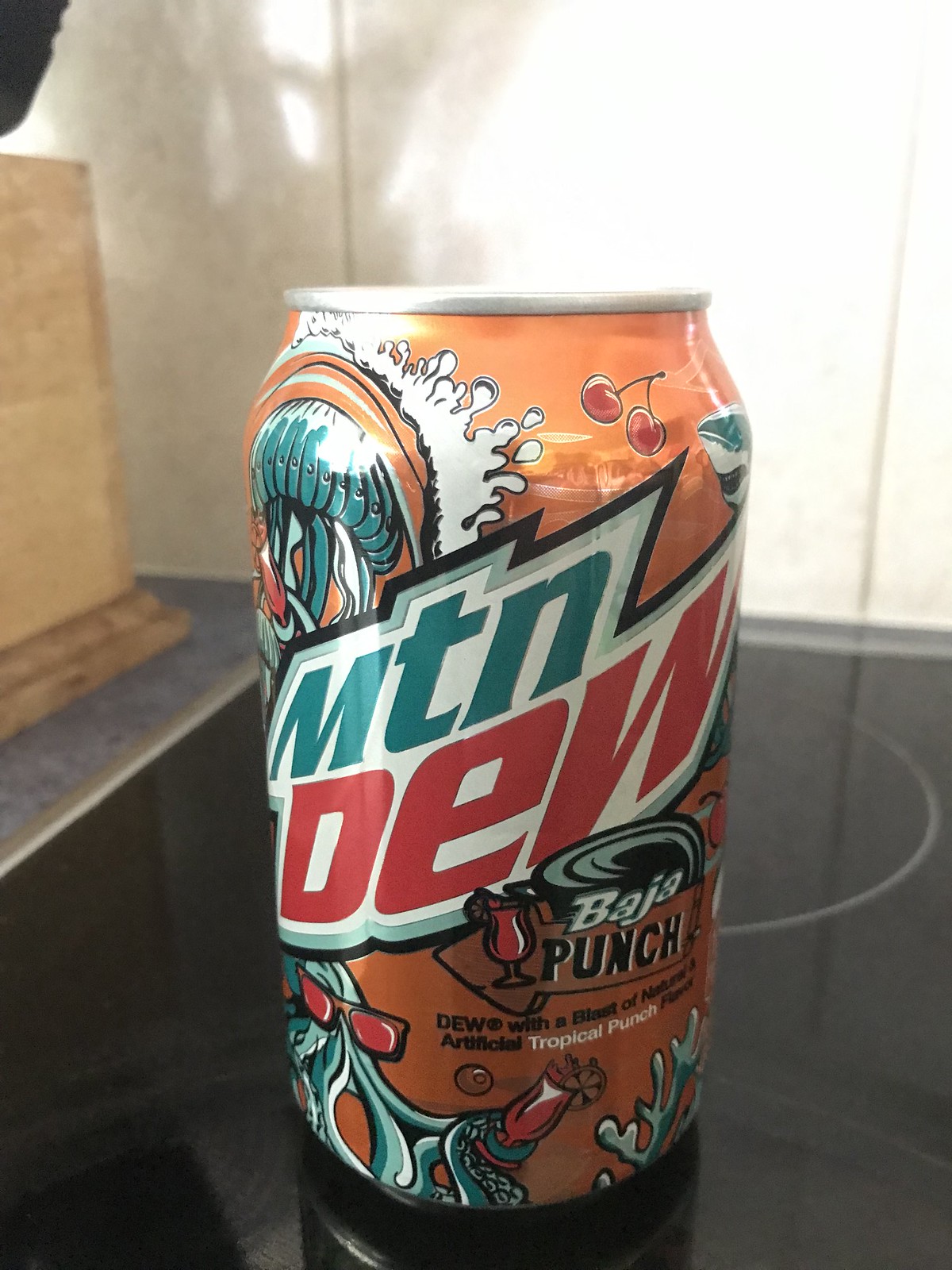The image features a prominently displayed can of Mountain Dew Baja Punch in a vertical rectangular format. The can, predominantly orange with a silver top, is adorned with vibrant and intricate designs. The brand name "Mountain Dew" is prominently placed at an angle, with "MTN" in green and "DEW" in red, slanting towards the upper right of the image.

Towards the bottom right of the can, there is a playful illustration of an octopus wearing sunglasses, holding a glass filled with a red tropical punch and garnished with an orange slice. Below the "Mountain Dew" logo, the words "Baja Punch" appear, accompanied by a small image of the same tropical punch glass held by the octopus. In addition, the text "tropical punch" is partially legible.

In the upper left section of the can, another whimsical creature, possibly a squid, can be seen. Meanwhile, the upper right section of the can features the face of a shark, adding to the dynamic and colorful design of the can. The entire illustration exudes a fun, tropical vibe, characteristic of the Baja Punch flavor.